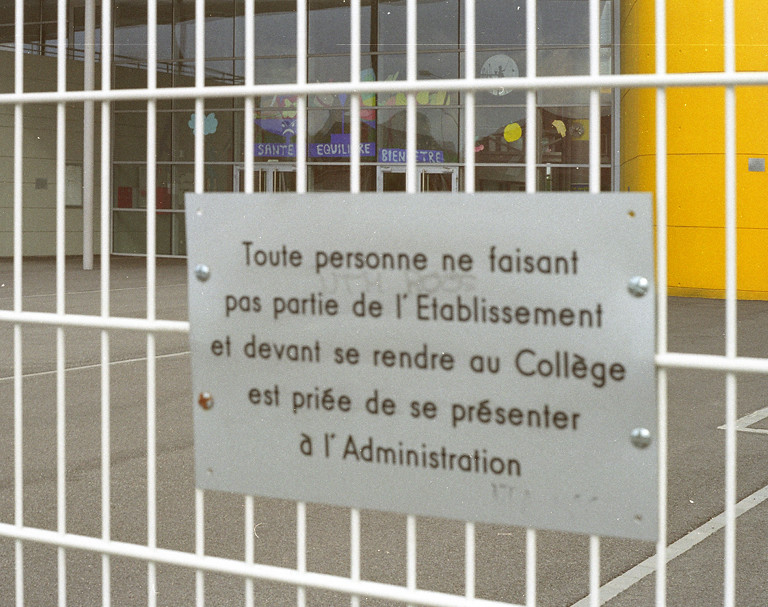This detailed photograph depicts a blurry image of a metal sign affixed to a white bar-type fence or gate, possibly by screws or adhesive. The sign is in a different language, likely French, with partially legible phrases such as "Devon say Rondray," "our college collage," and "pre days print Center." This suggests the location might be the front entrance to a college or an administrative center. Behind the fence is an entrance to what appears to be a classroom or similar room, characterized by a visible clock and a blue and white sign that reads "Sante aquilere be interest," though its exact meaning is unclear. The overall scene is devoid of people, and there is no date or additional text present. The gate seems to indicate a restricted or controlled access area, with multiple colors visible in the background, hinting at a lively environment, possibly an entertainment or educational facility.